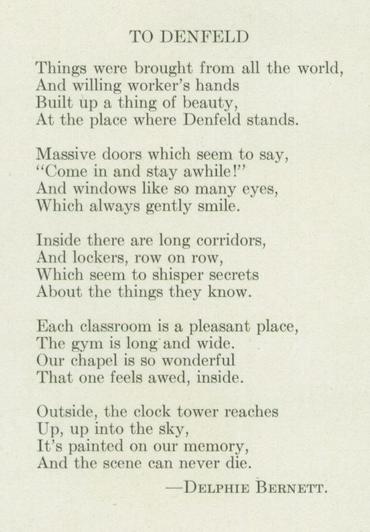This is an image of a poem printed on cream-colored, off-white paper with light black text, suggesting it might be from a book. The image is in portrait mode, making it rectangular and taller than wide. Centered at the top is the title "To DENFELD," followed by the author's name, Delphi Burnett, at the bottom. The poem is structured into five paragraphs and begins with, "Things were brought from all the world, and willing workers' hands built up a thing of beauty at the place where DENFELD stands." The description highlights massive doors that seem to invite people in and windows that appear to be smiling eyes. It continues by describing the interior's long corridors and rows of lockers, which "seem to whisper secrets" about their experiences. Each classroom is noted as a pleasant space, the gym is portrayed as spacious, and the chapel so inspiring that it leaves visitors in awe. The final lines depict the clock tower reaching towards the sky, vividly etched into one's memory, with the poem ending on the note that "the scene can never die."